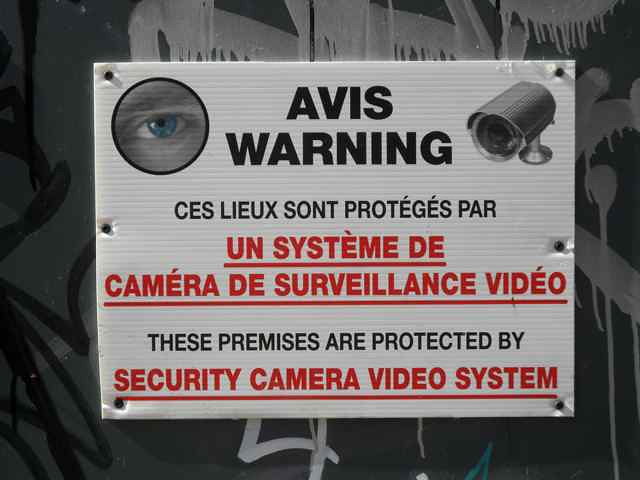The image depicts a warning sign affixed to a black-and-white graffiti-covered wall. The sign features a prominent header with the text "Avis Warning" in bold black letters. In the upper left corner, there's a circular image of a close-up eyeball, and on the upper right, there's an image of a security camera. Below the header, the text continues in French, "Ces lieux sont protégés par," followed by a bold, red underlined statement "Un système de caméra de surveillance vidéo." The English translation beneath reads, "These premises are protected by," with the phrase "Security Camera Video System" in red, underlined text. The white sign stands out starkly against the visually cluttered black and white graffiti background.